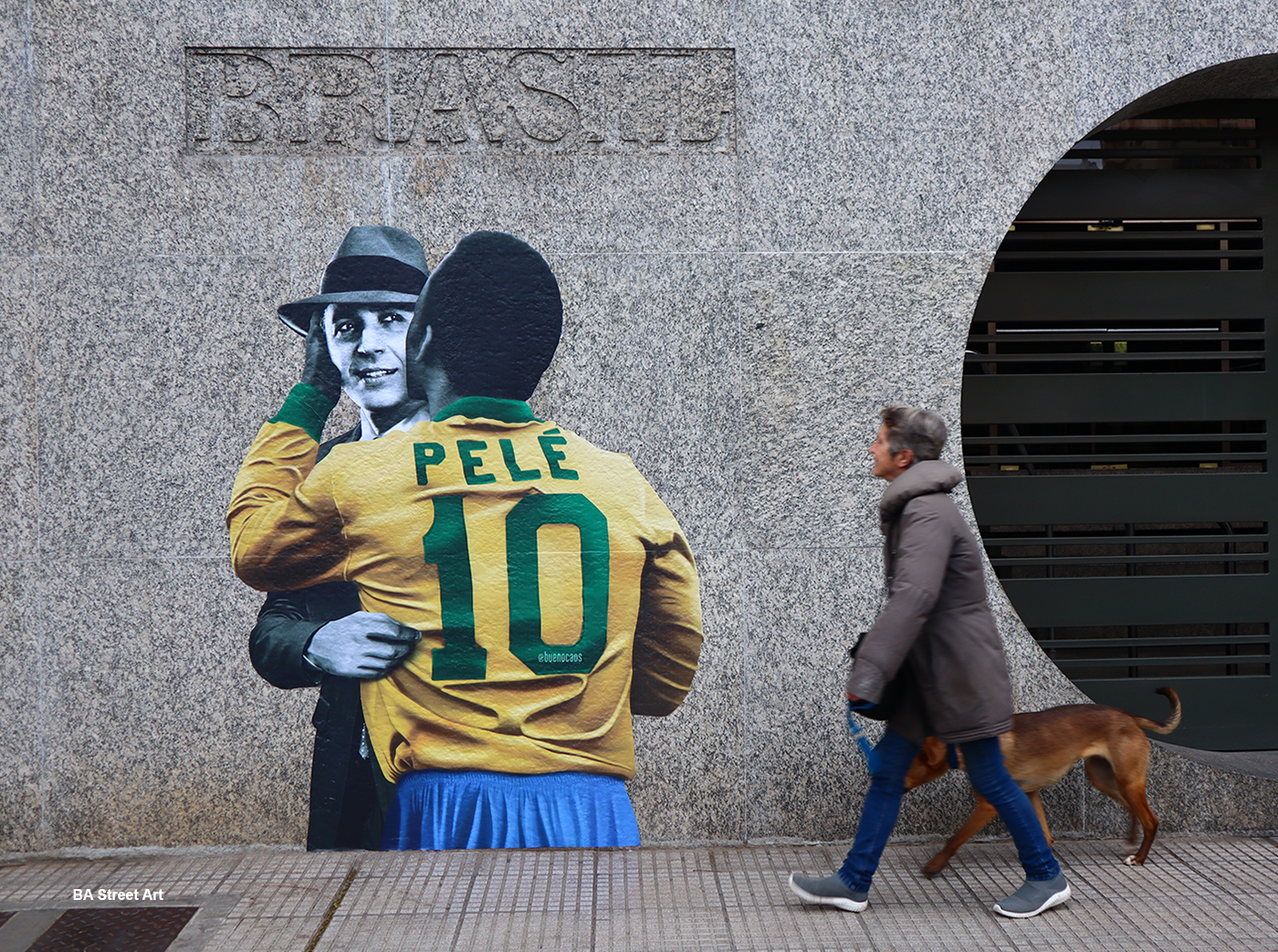The photograph captures a lively street scene, likely in Brazil, featuring a large stone wall with the word "Brasil" etched into it. Partially visible on the right side of the image is a semi-circular architectural cutout revealing black slats. Prominently displayed on the wall is a captivating mural blending elements of classic cinema and sports: a black-and-white depiction of Humphrey Bogart wearing his iconic fedora and suit, with his arm around Brazilian soccer legend Pelé. Pelé, dressed in a yellow and green jersey with the number 10 and blue shorts, leans in affectionately to kiss Bogart on the cheek, his hand gently placed on Bogart's face.

In the foreground, an older woman dressed in a gray winter coat, blue jeans, and gray sneakers walks along the sidewalk. She holds a blue dog leash attached to her brown dog, as she glances amusedly at the artistic tribute on the wall. The sidewalk beneath her is gray, and a metallic grate is also visible, adding texture to the urban landscape. This image beautifully contrasts the everyday with the culturally iconic, merging public art and daily life in an engaging outdoor snapshot.